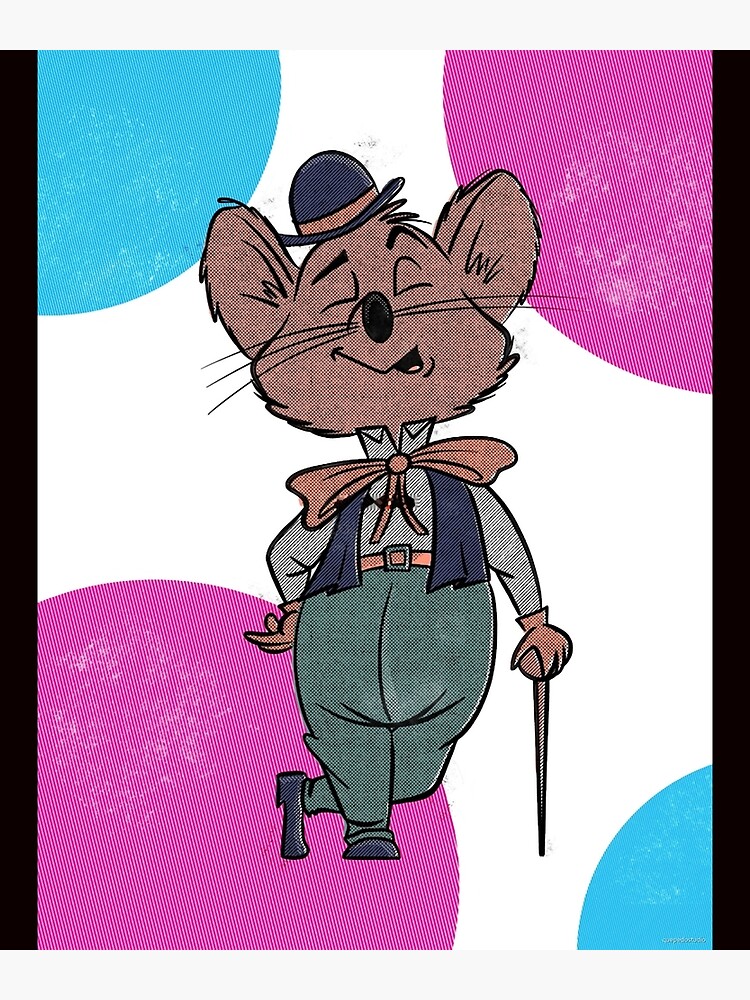A cartoon image depicts a finely dressed brown mouse wearing a small black bowler hat with an orange band, complemented by a matching orange bow tie beneath his slightly open mouth that hints at a whistle. His black whiskers and squiggly-marked ear hairs stand out prominently. He’s clad in a black-and-white striped shirt paired with green breeches, a bright orange belt with a square buckle, and gray dress shoes. The mouse's left hand holds a cane with a circular top, and his eyebrows are asymmetrical, with one straight and the other curved and lifted. He stands with one leg crossed behind the other against a background featuring a mix of pink and blue circles with visible textures. Specifically, there’s a large pink circle in both the top right and bottom left corners, a light blue circle in the top left corner, and a small blue circle in the bottom right corner, all framed by inch-thick black borders on the left and right sides.